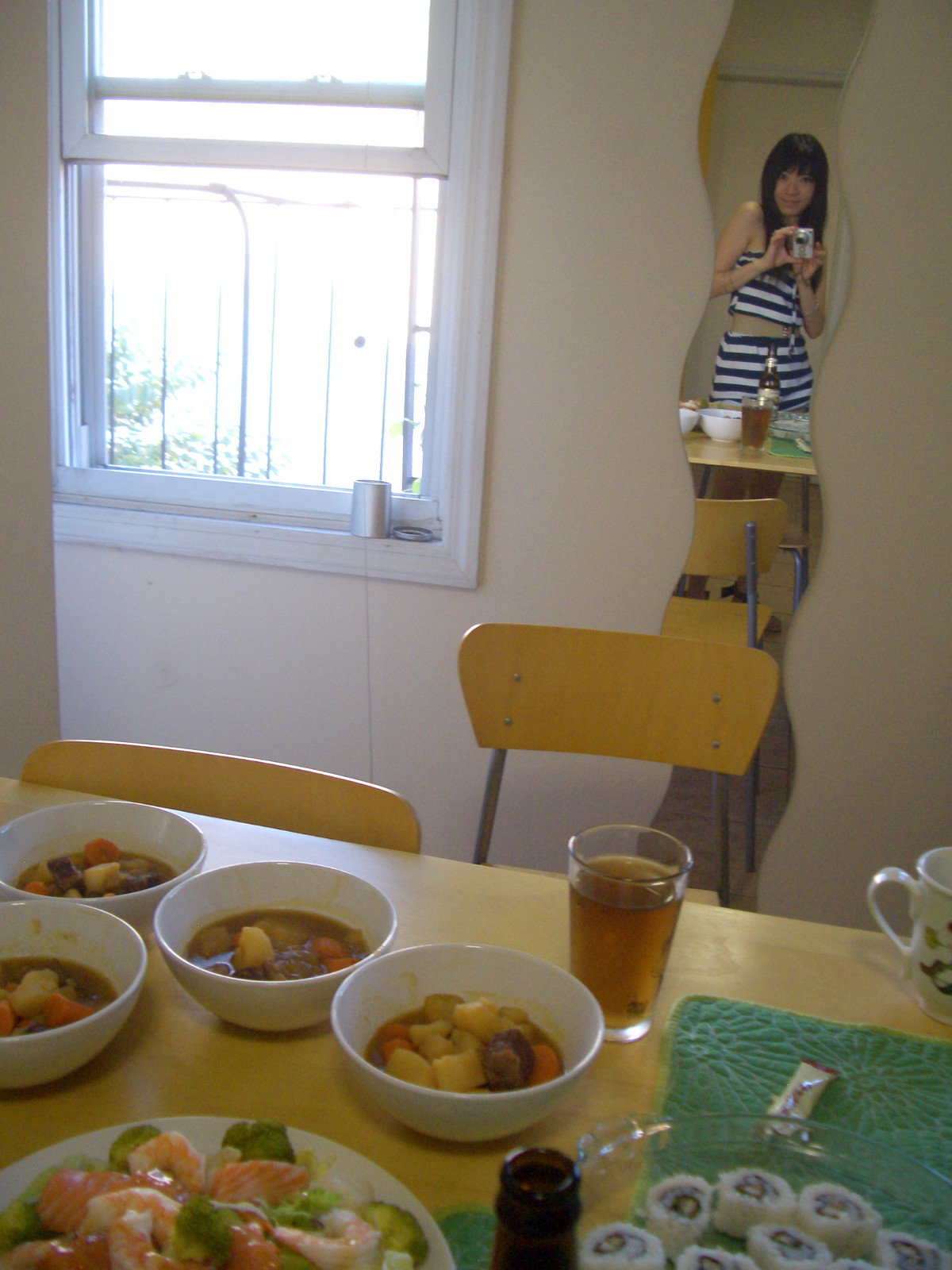This image appears to be taken inside a house, most likely in a dining room or kitchen. The foreground is dominated by a light tan or beige wooden table that is laden with various dishes and items. The table is crowded with a big round plate featuring food items, including vegetables, meat, shrimp, and sushi rolls. Four bowls containing food, possibly soups with potatoes, meat, and carrots, are also present. There is a glass filled with a brown liquid, possibly apple juice, and the top of a beer bottle is also visible. A chair is pulled out while another remains tucked in.

In the background, a white wall is visible, with a white-framed window on the top left, suggesting it is sunny outside. On the top right, a wavy mirror reveals the reflection of a woman taking a picture. She appears to be young, with long black hair and bangs, potentially of Asian descent. She is wearing a matching outfit consisting of a white and black horizontal striped top and bottom. Her reflection further reveals portions of the items spread across the table in front of her.